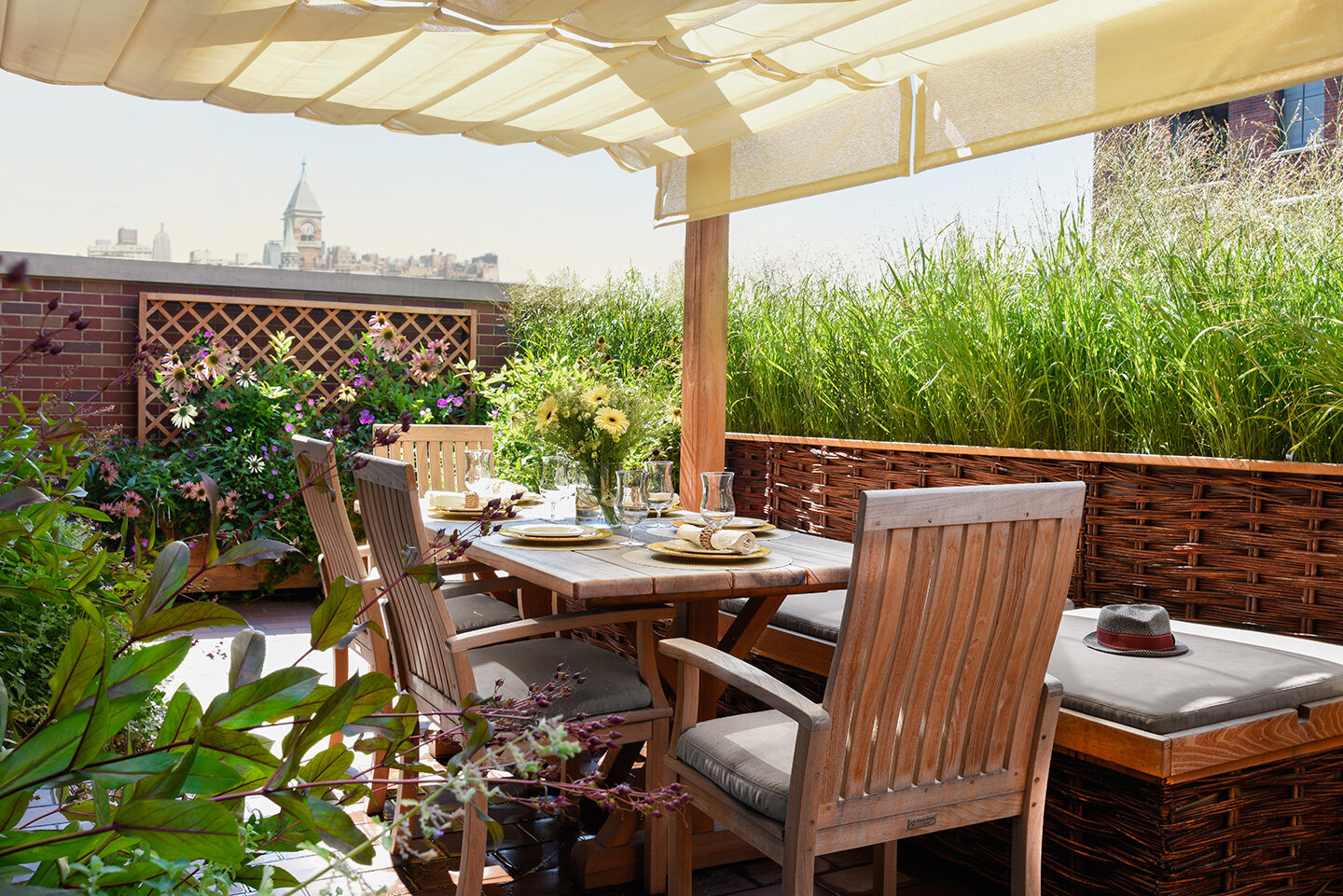The photograph captures a cozy outdoor patio restaurant set under a yellow canopy filtering sunlight onto the scene. At the center is a wooden table adorned with a vase of yellow and green flowers. The table is neatly set with ceramic plates, glass cups containing clear liquid, and napkins. Surrounding the table are a variety of seating options: four wooden chairs with backrests, two stool-like chairs without backrests, and a bench with gray cushions. To the right, a gray hat with a red band is placed on one of the stools. The background features a lush array of green plants, a brick area with lattice entwined with climbing plants, and distant multi-story buildings under a clear sky, completing the picturesque and serene ambiance.